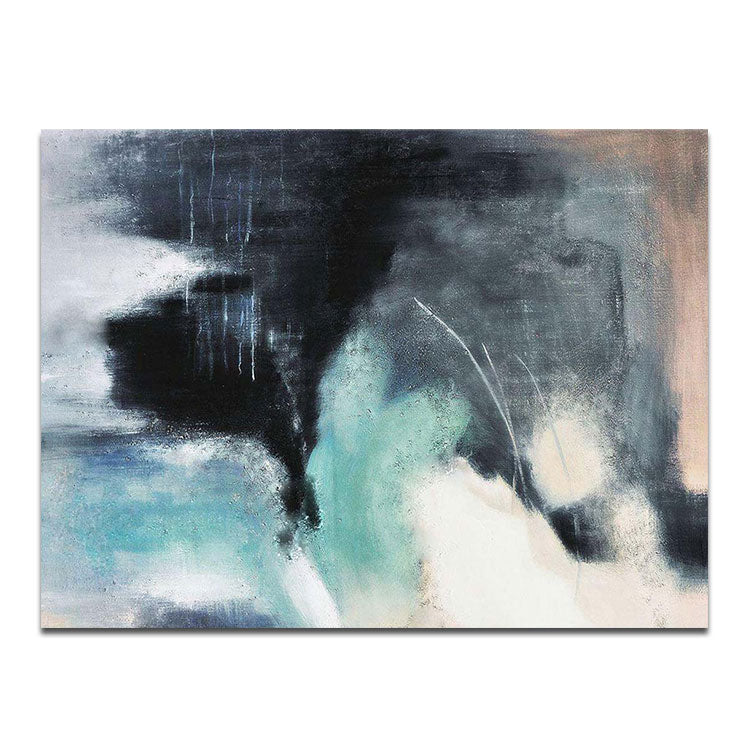The image captures an abstract piece of art, brimming with colorful and blended hues. Predominantly, you find shades of gray and black interspersed with turquoise, blue, white, beige, and cream, forming a cloud-like pastiche. The turquoise appears notably in the bottom left and central regions, while the gray and black dominate the top left and center right areas. This artwork, potentially created with watercolors on a painter's canvas, presents a smudged, blended appearance with no distinct shapes or written elements, resulting in a harmoniously chaotic pattern. Its horizontal layout and rectangular shape, combined with the evocative use of colors and textures, can even evoke images akin to a gray ship among clouds or smoke, adding a layer of interpretative depth.